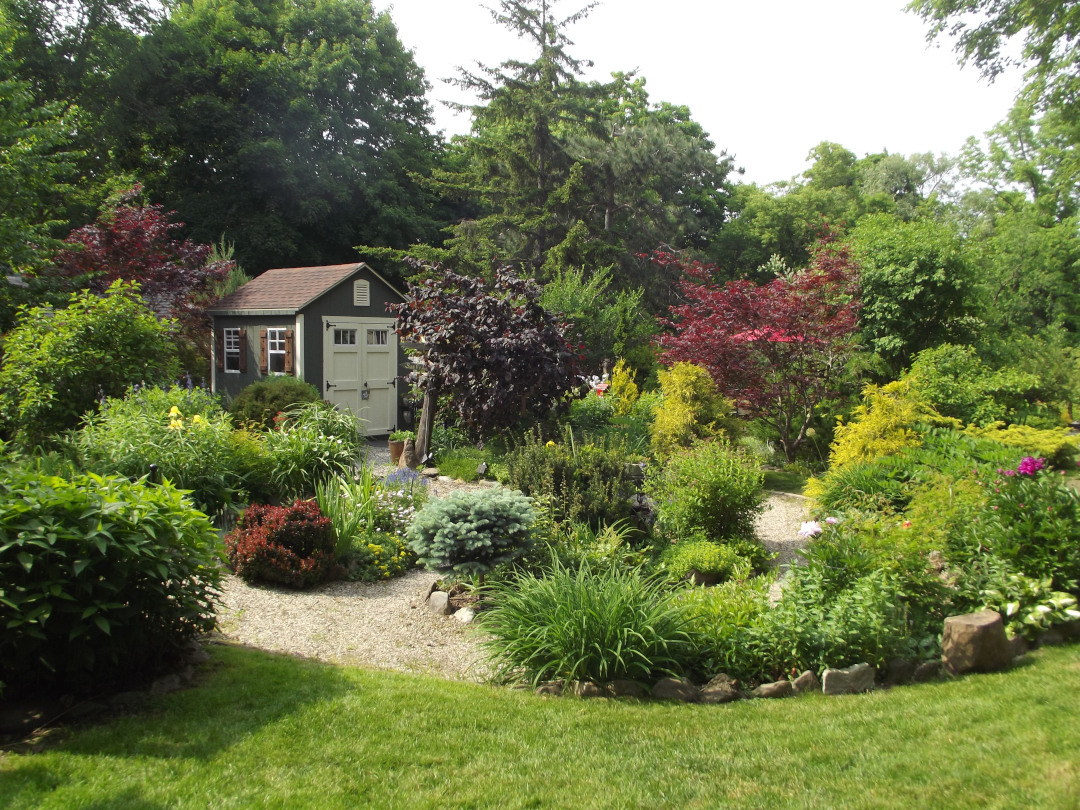The image captures a tranquil and well-manicured garden scene, exuding the lush vibrancy of summertime. At the center is a charming little shed painted in a dark olive green with white double doors adorned with black hardware, featuring three glass panes on each door. It has a brown shingled roof and two white framed windows with matching dark brown shutters. The shed is nestled amidst tall, diverse trees in the background under a clear blue sky.

In the foreground, a well-kept lawn leads to a varied landscape of shrubs and ornamental grasses in shades of deep purple, vibrant maroon, yellow, and red, some of which are flowering. A pebble-lined pathway meanders through the garden, bordered by larger stones marking different planting areas. Among the green and multicolored foliage, there are noted flower beds and a possible hint of lavender, adding to the garden's aesthetic and sensory appeal. A tree stump and an inviting birdhouse add quaint touches to the scene. This picturesque garden, possibly part of someone's elaborate backyard, radiates beauty and tranquility, making it both visually appealing and serene.